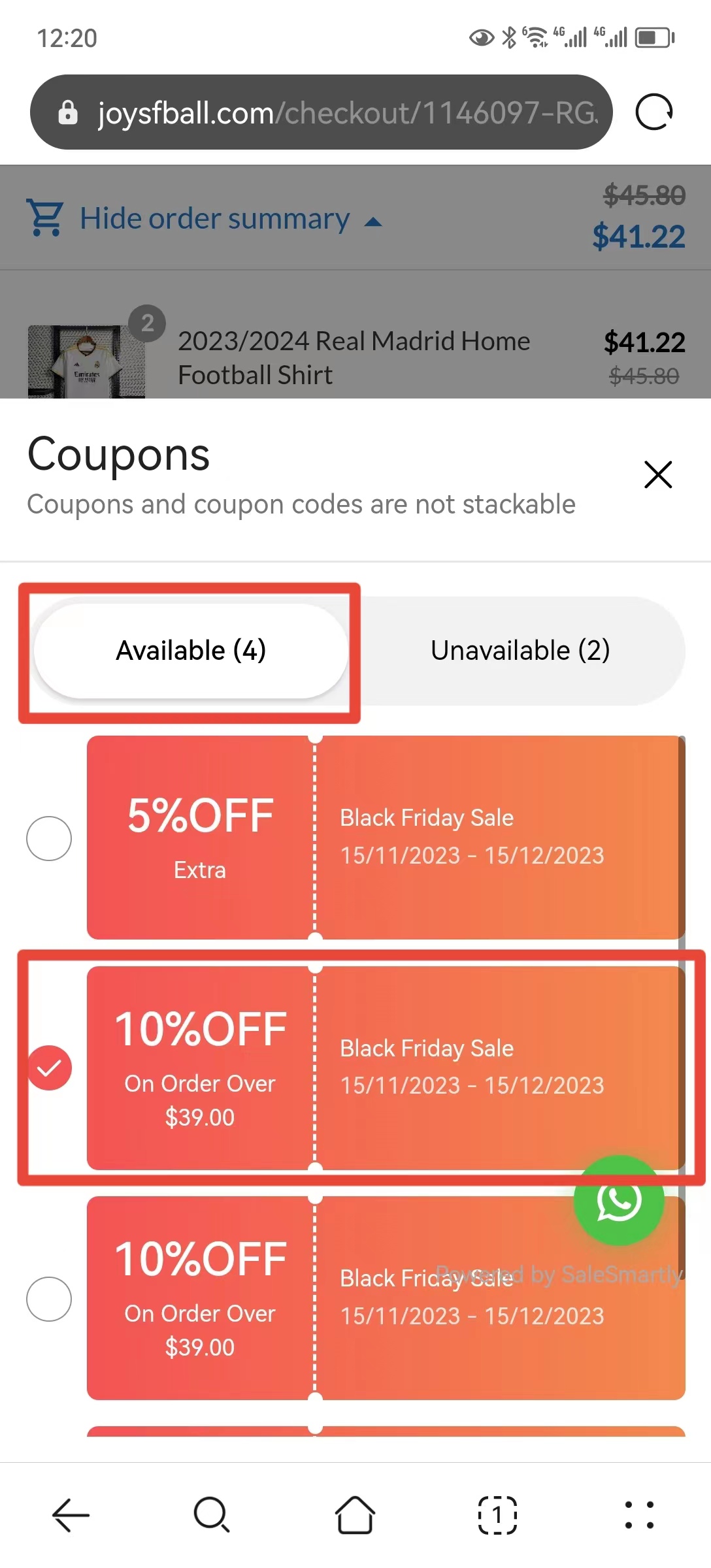This screenshot captures a device screen displaying a webpage. At the top left corner, the device shows the current time as 12:20. On the top right, various status bar icons are present, including the Bluetooth icon, Wi-Fi signal icon, 4G indicator, SIM 1 and SIM 2 icons indicating full network reception, and a battery icon showing approximately half charge.

Below the status bar, a URL is visible: joyosfball.com/checkout/1146097-ROG. The main content of the page shows a high-level summary, with the price prominently displayed as $41.22. The item being highlighted is the "2023-2024 Real Madrid Home Football Shirt." Additionally, a notification regarding the availability of coupons is mentioned, stating "coupons available for unavailable tour," although the exact meaning is unclear from the context provided.